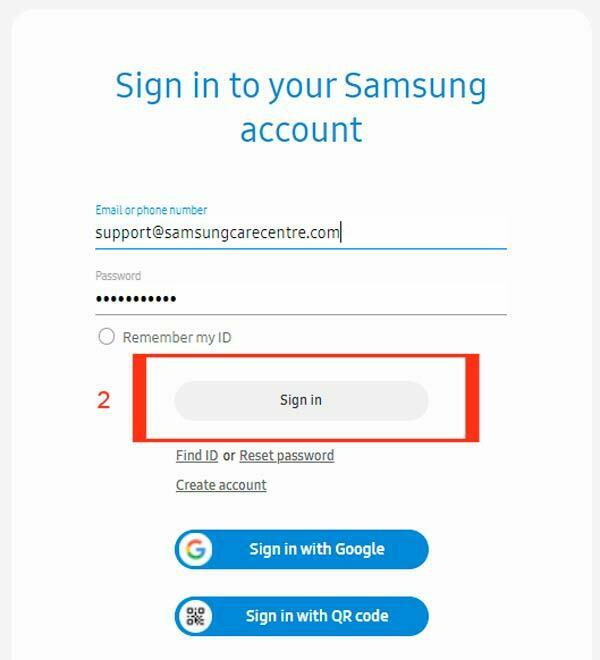The image depicts a Samsung account sign-in page on a white background. At the top, in blue text, the header reads "Sign in to your Samsung account." Below this, also in blue text, is a label for "Email or phone number" with the text box below it filled in with "support@samsungcarecenter.com." Next, there is the word "Password" indicating a text box for password entry, which is filled with hidden characters for security.

Beneath the password box, there is an unchecked circle labeled "Remember my ID." Directly below this lies a rectangular red-bordered box with a red number "2" beside it, containing the text "Sign In."

Underneath this box, there are three hyperlinked options sequentially listed: "Find ID," "or Reset password," and "Create an account." Further down, on a blue background, there is the Google symbol followed by white text reading "Sign in with Google."

After a blank white space, another blue background appears, featuring a QR code symbol next to white text that says "Sign in with QR code." The rest of the page beneath this section remains blank.